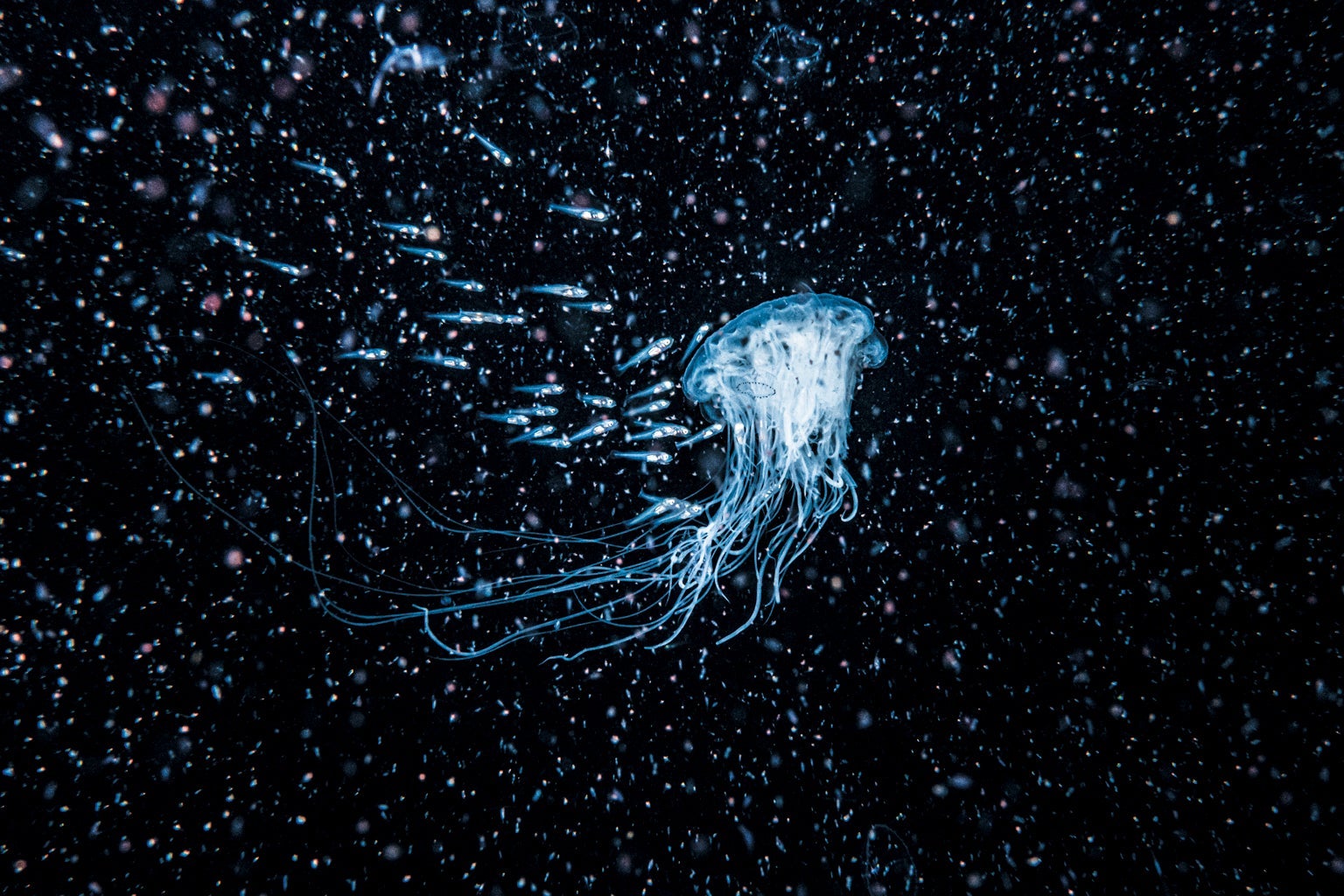This image depicts an ethereal, almost celestial scene, characterized by a luminous blue jellyfish with long, flowing tendrils that curve gracefully towards the upper left corner. Surrounding the jellyfish is a small school of neon blue fish, numbering around 15 to 20, clustering together and swimming towards the vibrant, glowing jellyfish at the center. The black background is speckled with tiny dots of blue, purple, and pink, giving an impression of an underwater space filled with tiny, luminescent particles, possibly plankton. These specks vary in focus, adding depth and a sense of motion to the scene. The overall effect is a mesmerizing contrast between the bright, glowing subjects and the dark, expansive void, resembling an alien landscape in the deep sea.